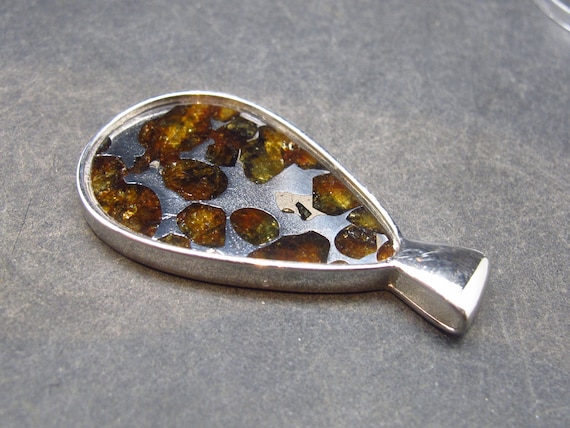This is a color photograph showcasing a teardrop-shaped pendant dish that resembles a decorative piece possibly in the process of being constructed. The dish, which appears to be made of silver, features a sleek, shiny, metallic finish with a knob-like taper at one end, contributing to its overall elegant design. The interior of the dish exhibits a grainy, shiny and viscous substance interspersed with amber-colored crystal-like chunks, lending a striking contrast against the smooth silver surface of the dish. The amber elements vary in shape, appearing as both irregular blobs and more defined oval pieces. The dish is set on a gray, granite-like surface with white lines running through it, further enhancing the sophistication of the image.